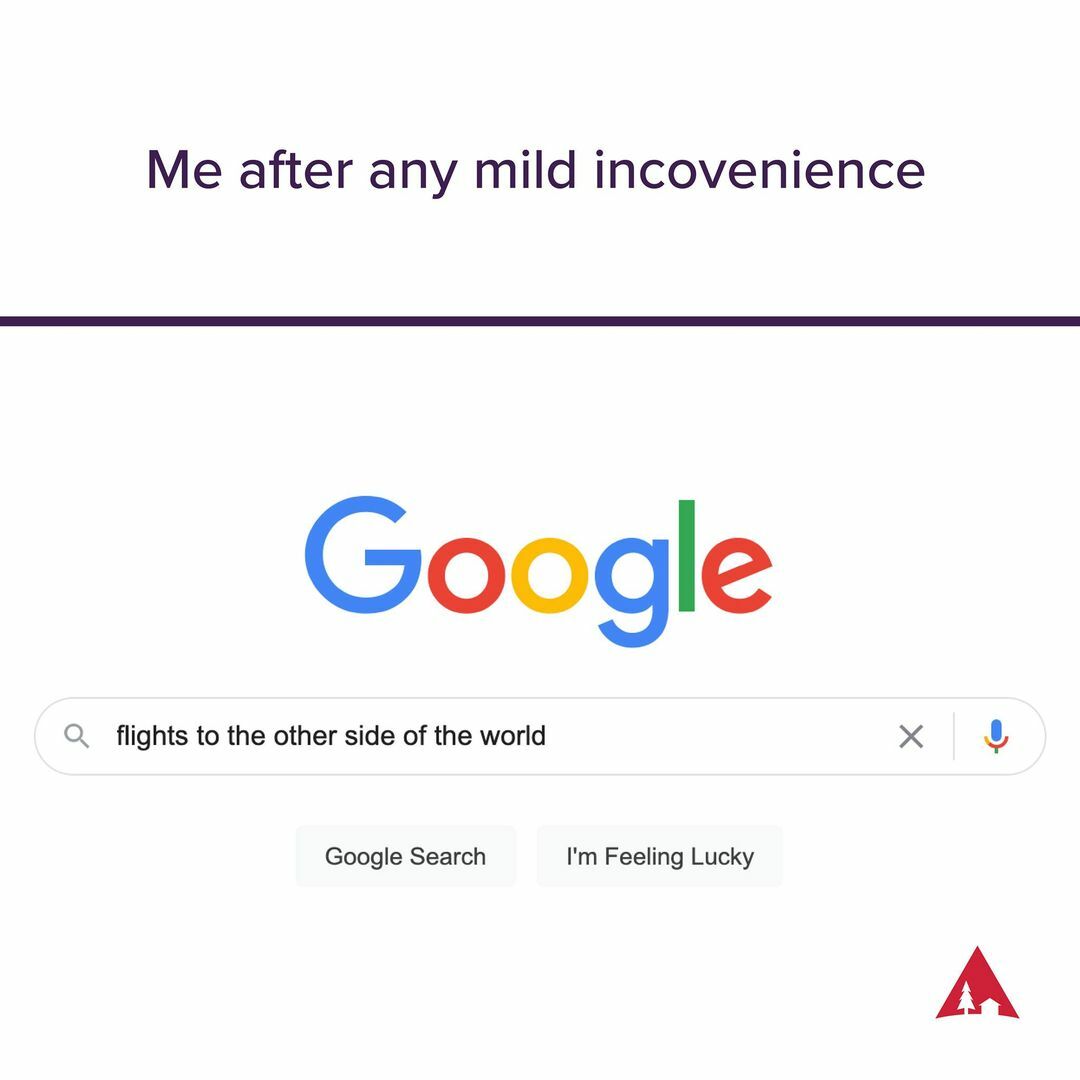This meme features a clean, white background divided into two sections. The top half contains a humorous caption in a prominent, clear purple font that reads, "Me After Any Mild Inconvenience." Below this caption is a thicker purple dividing line that neatly separates the sections.

The bottom half of the meme is a screenshot of a Google search page. The iconic Google logo is presented at the top with its familiar color scheme of a blue "G," red "O," yellow "O," blue "G," green "L," and a red "E." The search bar, centered in the white space, contains the gray magnifying glass icon followed by the typed query, "Flights to the Other Side of the World," with a small "X" to clear the input on the right. To the far right of the search bar is a blue and red microphone icon.

Below the search bar, the customary Google search elements are displayed. The "Google Search" button is depicted with gray text inside a white button outline, and to its right, the "I'm Feeling Lucky" button is similarly styled.

A small, unfamiliar red triangle icon featuring a white tree and house is positioned below these buttons, adding an unusual and eye-catching element to the image.

Overall, the symmetrical layout and light-hearted content aim to amuse viewers with its relatable and exaggerated depiction of seeking an escape in response to minor inconveniences.